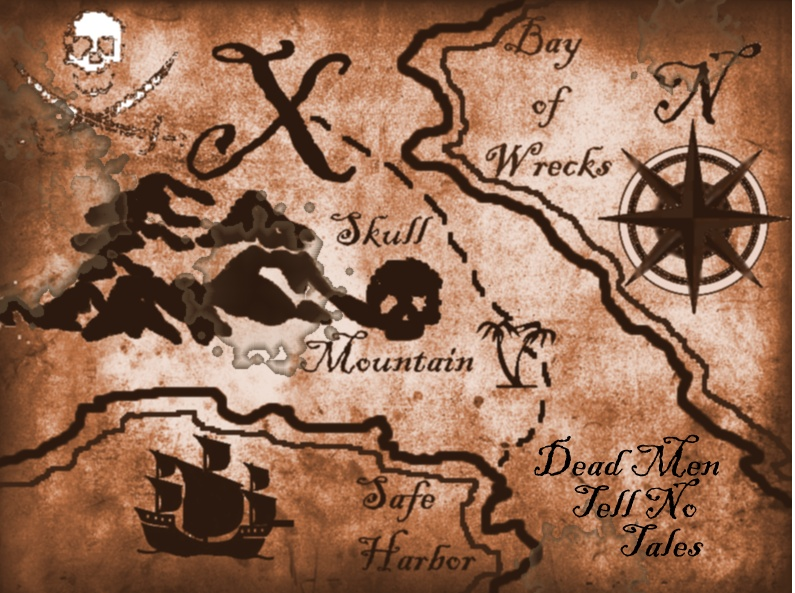The image is a detailed, rectangular pirate map measuring about six inches wide and four inches high, rendered in tones of tan and reddish-brown with black outlines. The map appears aged, with dark brown watermarks staining the borders, enhancing its antique look. In the upper left corner, a white skull with two crossed swords beneath it forms an X, evocative of pirate symbolism. Nearby, there's a large X marking the treasure spot, accompanied by a dotted line leading to it. The map also features a compass rose prominently in the upper right corner with "North" labeled at the top and the words "Bay of Wrecks" situated next to it.

In the map's center, "Skull Mountain" is marked with a small, menacing skull icon, partially obscured by clouds. The outlines of the land are depicted as curving lines that might represent rivers or the coastline. The lower left corner shows a multi-sailed ship labeled "Safe Harbor" sailing in what appears to be a water area. The bottom right corner bears the ominous inscription, "Dead Men Tell No Tales." Adding to the visual lore is the image of a lone palm tree somewhere on the map. The entire scene is imbued with a sense of adventure and mystique, reminiscent of an artifact from a pirate saga like "Pirates of the Caribbean."